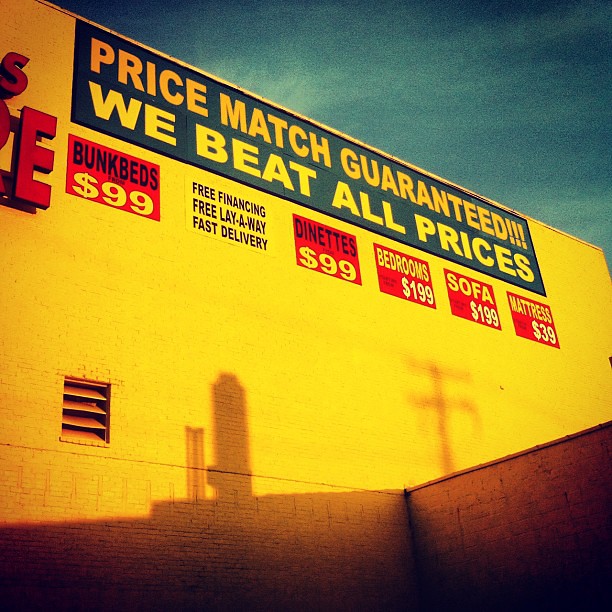This outdoor photograph, taken at an angle from street level, captures the side of a large yellow brick building under a blue sky punctuated by a few white clouds. The image prominently features several signs on the wall of the building. The main blue rectangular sign at the top reads "Price Match Guaranteed!!!" in yellow capital letters, and just below it, "We Beat All Prices" in white capital letters. Further down the wall, there are a series of smaller rectangular advertisements: the first on the left features "Bunk Beds $99" in red text, followed by "Free Financing, Free Layaway, Fast Deliveries" in black text. Other signs include "Dinettes $99," "Bedrooms $199," "Sofas $199," and "Mattresses $399." Additionally, the photograph shows a vent with three horizontal slats on the lower left side and a partial red sign with the letters "S" and "E" in the upper left corner. The image highlights the detailed advertisement display against the backdrop of a setting sky, adding a dynamic and realistic touch to the scene.